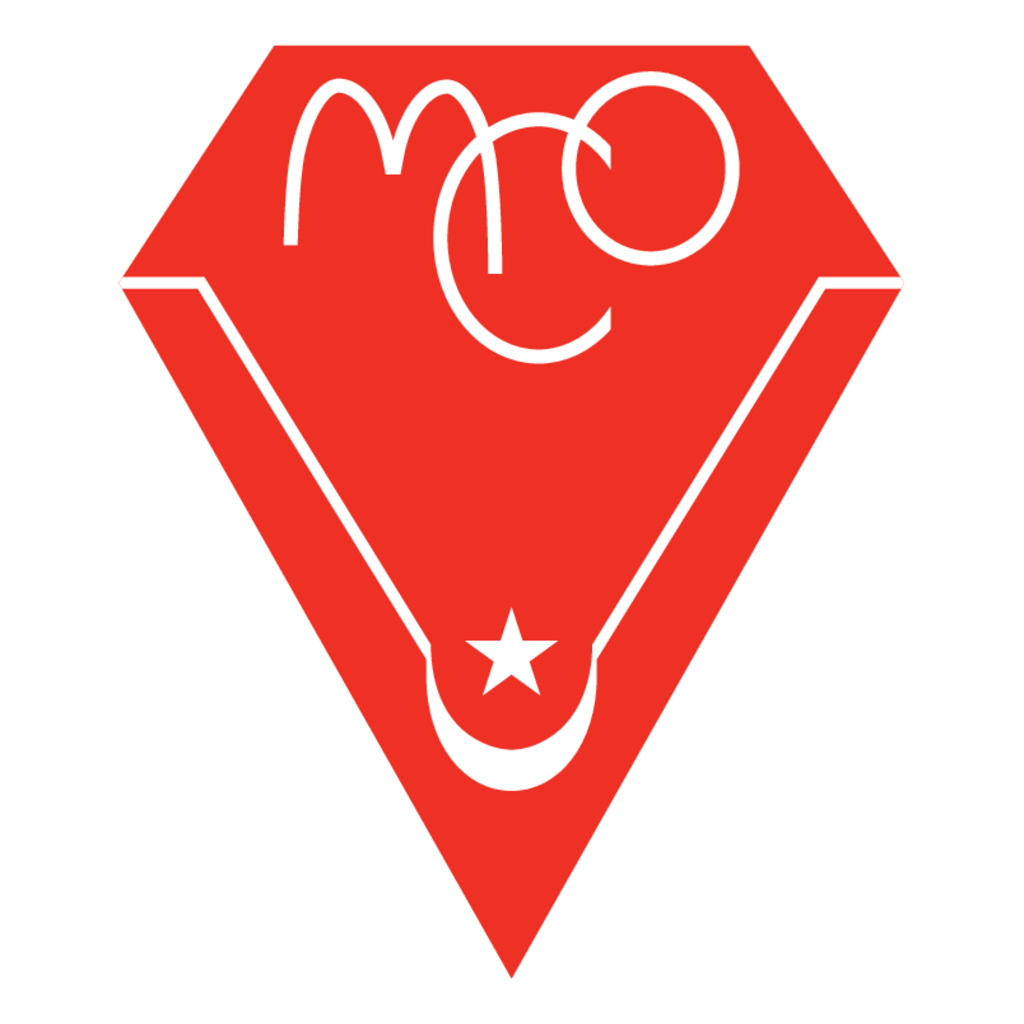The image features a prominent logo set against an all-white background, depicting a large red diamond shape that dominates the frame. Inside the diamond, at the top, there is white text reading "MCO," with the "M" resembling the iconic McDonald’s logo and the "C" appearing larger and not overlapping with the other letters in the middle. Below the text, the diamond contains a downward-pointing design element that forms a V-shape, with a sharp point at the bottom. Additionally, there is a white star and crescent moon at the bottom of the diamond, the moon pointing upwards. The logo's design and bold red and white color scheme give it a versatile and professional appearance, suggesting it could be used for a company's branding, such as on a business card, website, or company presentation.